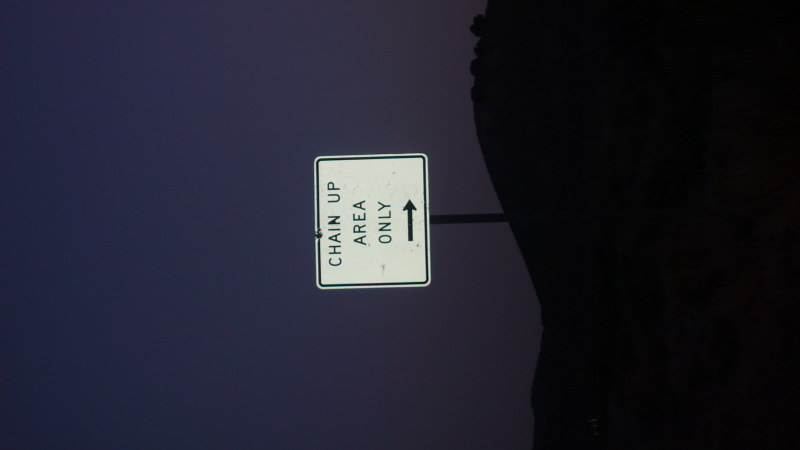The photograph, likely taken at night, is presented sideways and features distinct sections with a dark blue background on the left transitioning into a purely black background on the right. These backgrounds are divided by a curvy, vertical line approximately 40% from the right edge. Dominating the center of the image is a white sign with black letters saying "Chain Up Area Only," and an arrow initially directed to the right, now pointing upwards due to the image's 90-degree rotation counterclockwise. The sign is fixed to a black horizontal rod situated on the right within the dark black backdrop. The black area suggests the presence of a hill or ridge, perhaps with tree outlines faintly visible at the top, enhancing the photo's outdoor nighttime setting.